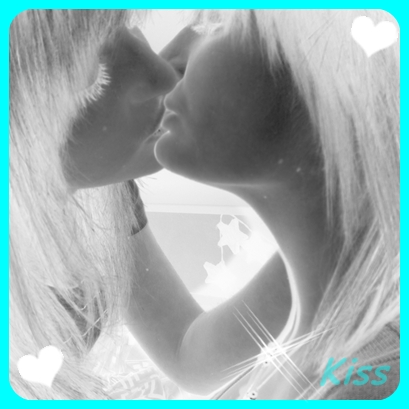The image depicts a black-and-white reverse negative stylization of two girls about to kiss. Their faces are close, with features blurred and scarcely distinguishable due to the high contrast that swaps the usual light and dark values — their skin appears dark while their hair and eyelashes are stark white. Both have long, straight, spiky hair, and the girl on the left has her arm bent, gently resting on the right girl's shoulder. The photograph is surrounded by a neon teal border with additional elements: a white heart in the upper right and lower left corners, and the word "kiss" written in the same teal color in the bottom right corner.